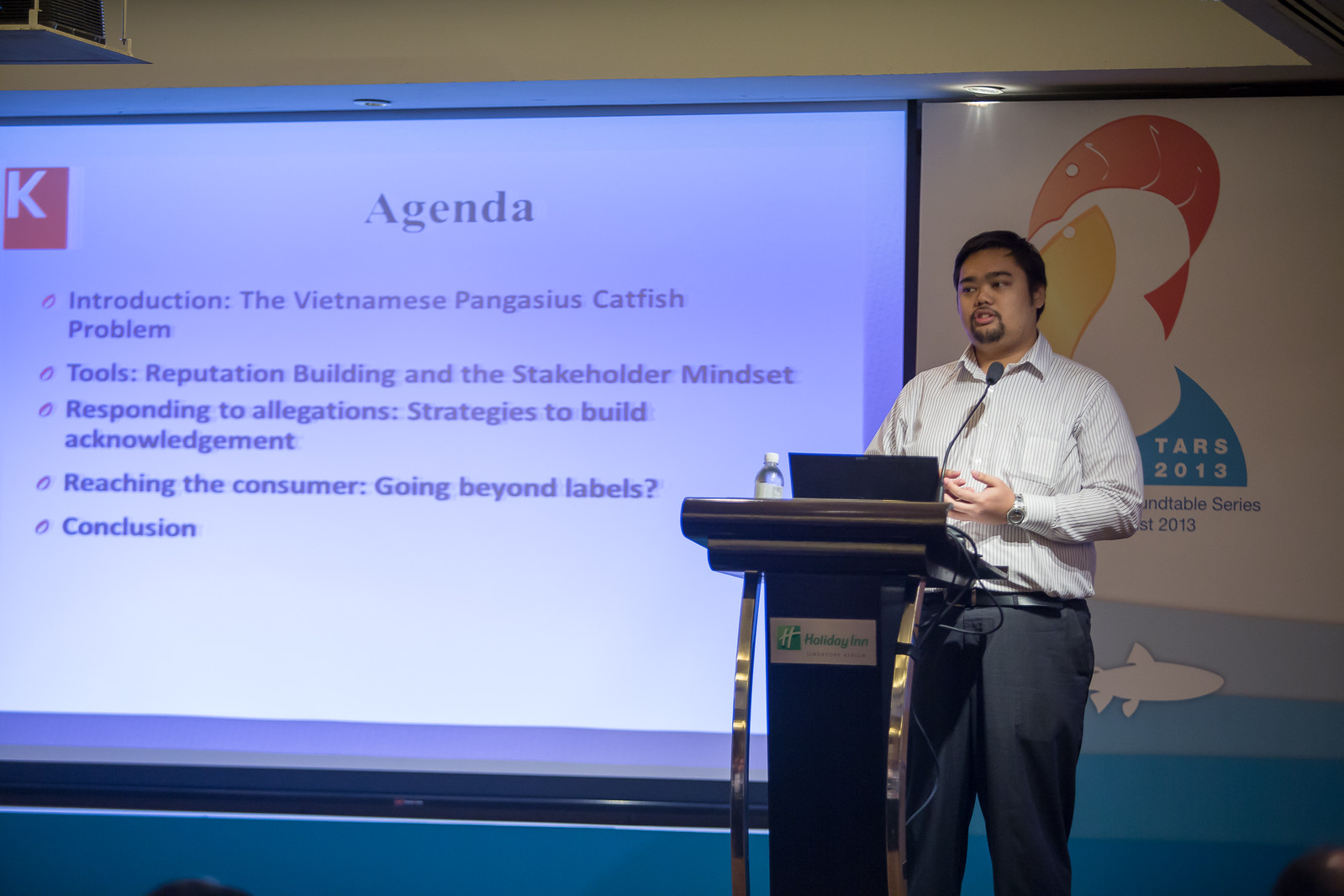The image depicts a man speaking at a conference held at a Holiday Inn. He has tanned skin, short black hair, and a short beard, and is dressed in a striped white and blue shirt paired with navy blue trousers and a black belt. He stands behind a small podium with a microphone and a laptop on it, alongside a bottle of water. To the left, there's a white screen displaying a detailed agenda for his presentation. The agenda is divided into five parts: "Introduction to the Vietnamese Pangasius Catfish Problem," "Tools, Reputation Building, and Stakeholder Mindset," "Responding to Allegations, Strategies to Build Acknowledgement," "Reaching the Consumer, Going Beyond Labels," and "Conclusion." Behind the speaker, there appears to be a logo related to wildlife from the year 2013, signifying the conference's theme.